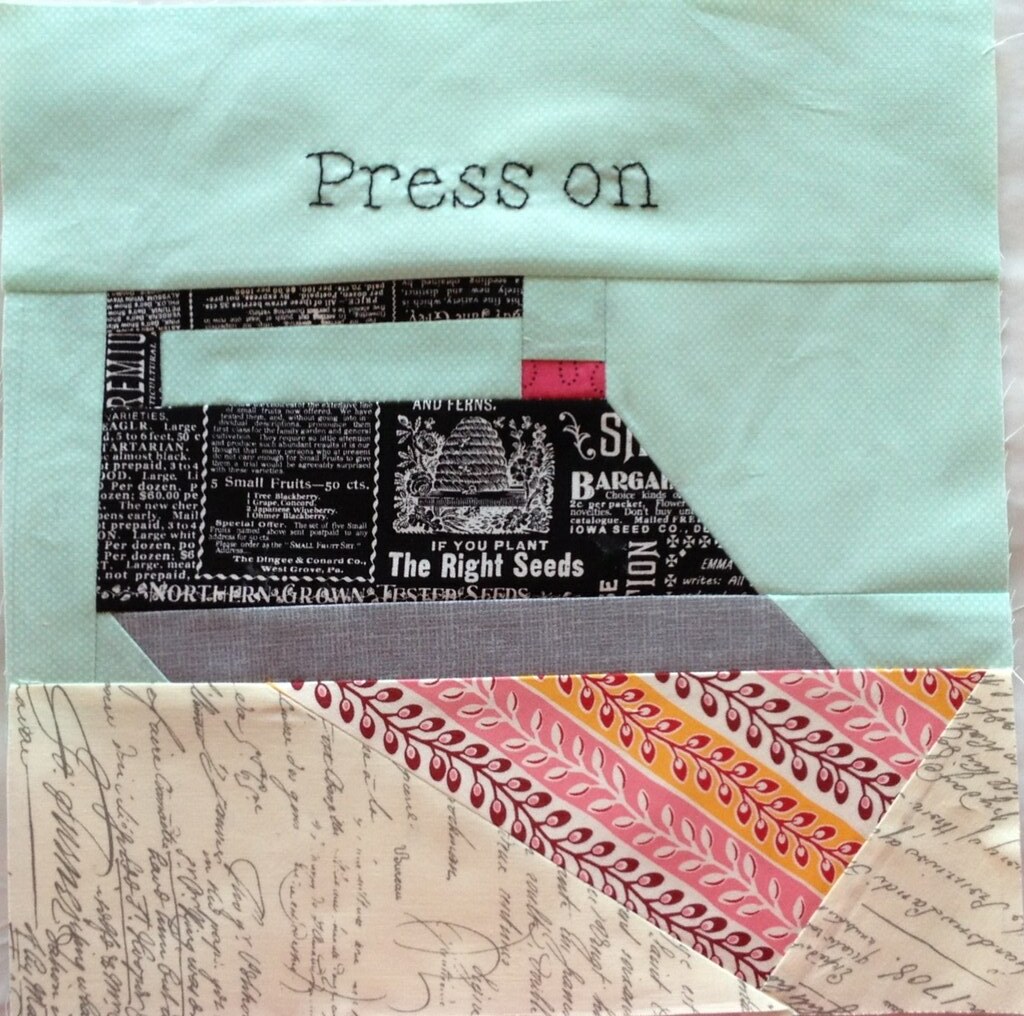The image depicts a handmade fabric collage laid on a plain white background that fills the entire frame. The intricate design features several pieces of fabric intricately stitched together, incorporating both rectangular and angled shapes. The top row is light green and includes the embroidered text, "PRESS ON." Below, a mix of various fabric pieces is stitched together, dominated by the same green fabric at the top, interspersed with a central black piece resembling old newspaper clippings. Toward the bottom, there's a light tan fabric reminiscent of aged parchment, adorned with calligraphy and signatures, giving it the appearance of an old letter. Adding a vibrant touch, there is fabric featuring a repetitive pattern of vines in red, pink, and white, each set against contrasting backgrounds of white, pink, and yellow respectively. This eclectic combination of textures and colors—from off-white, light blue, gray, and maroon to patterns of pink and red vines—creates a rich, visually engaging piece, possibly crafted in an arts and crafts setting.